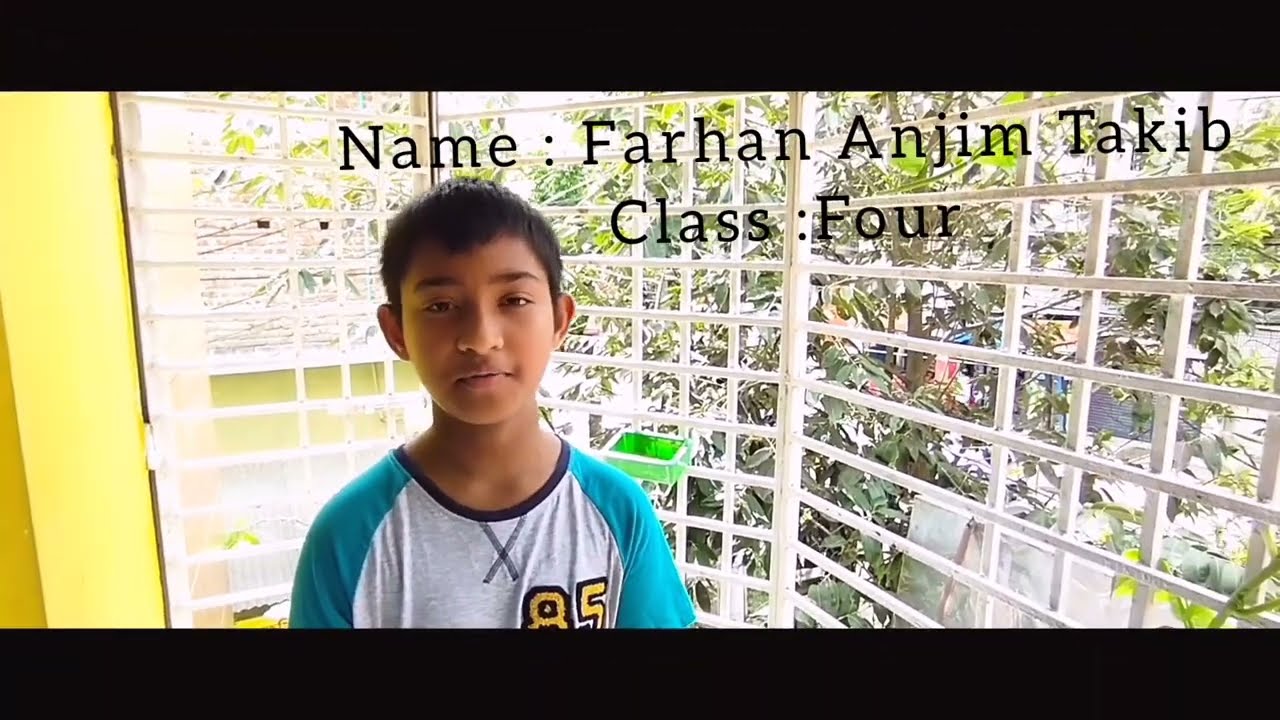This photograph features a young boy of Asian descent, centered and facing the camera. The image captures him from his chest up, showcasing his dark hair and dark eyes. He is dressed in a t-shirt with light blue sleeves and shoulders, and a gray chest area emblazoned with the number "85" in yellow with a black outline. Above the boy's head, the text "Farhan Anjum Takib, Class 4" is printed in black against a black horizontal strip. Behind the boy, there is a large window with white criss-cross bars, allowing a view of trees and other buildings outside. To the left of the boy in the background, a yellow painted wall can be partially seen, along with a small green rectangle hanging from the lattice work. The top and bottom of the image are bordered by black horizontal strips.